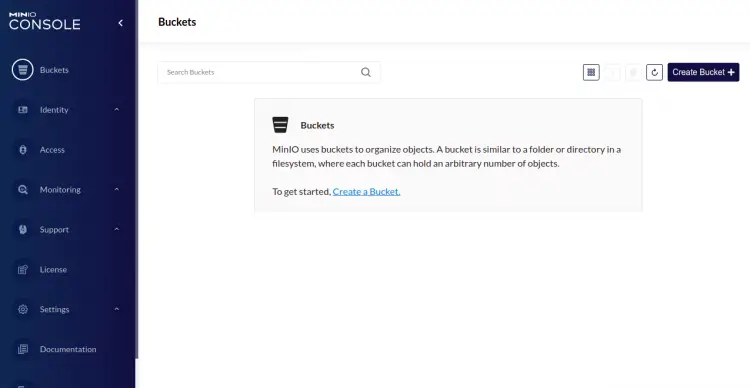This image is a detailed screenshot of the MinIO Console interface, designed for managing object storage. The console features a dark navy blue scheme, almost black, contrasted with white font for readability. 

On the left side, a vertical navigation menu displays a series of icons and labels for different tabs, including Buckets, Identity, Access, Monitoring, Support, License, Settings, and Documentation. Currently, the selected tab is "Buckets."

The main section under the "Buckets" tab contains a prominent heading labeled "Buckets." Directly below this heading, there's a search bar with the placeholder text "search buckets" and an accompanying magnifying glass icon. 

Beneath the search bar, a large gray rectangle provides additional details. It features a bucket icon beside a description that reads: "Buckets: MinIO uses buckets to organize objects. A bucket is similar to a folder or directory in a file system where each bucket can hold an arbitrary number of objects. To get started, create a bucket." The phrase "Create a bucket" is highlighted in blue, suggesting it is a clickable link.

In the top right corner of the main section, there is a prominent button labeled "Create Bucket" accompanied by a plus sign, inviting users to create a new bucket.